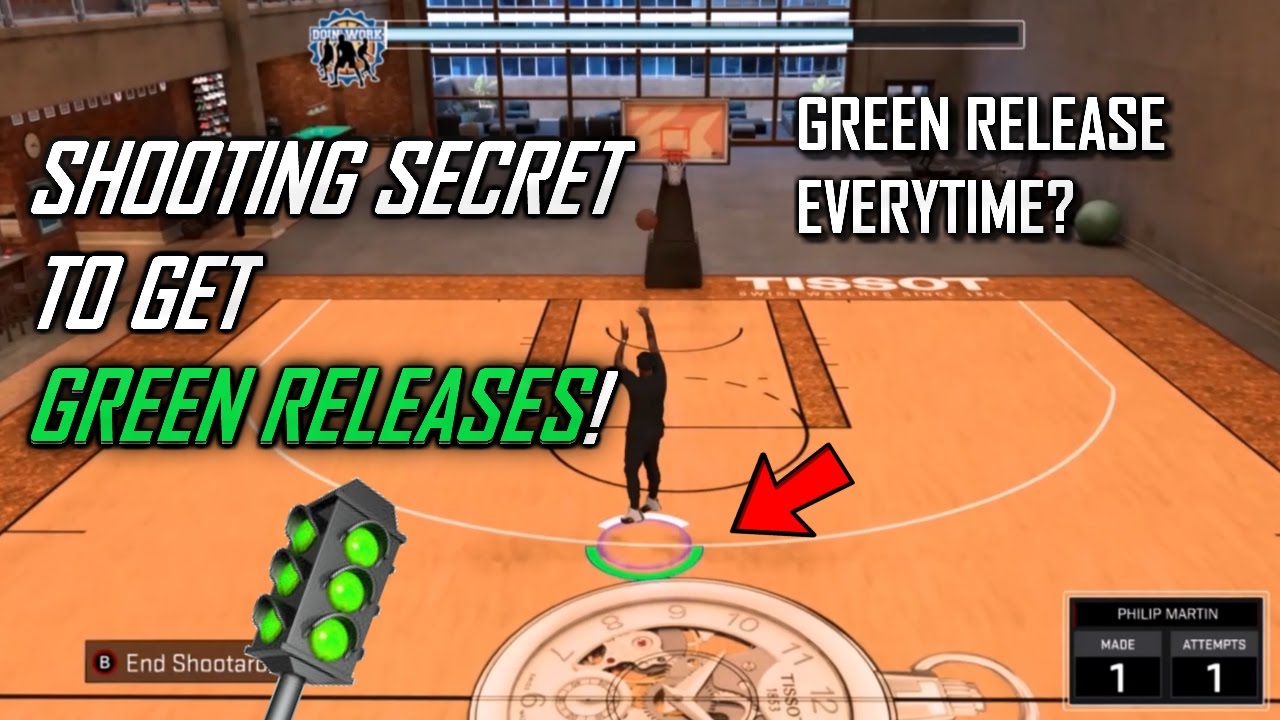This image depicts a detailed scene from a basketball video game set inside a gymnasium. The gym’s background features intricately described elements, starting from the right side with a brown wall that extends upward and outward from the corner, running horizontally almost an inch before six windows appear. These windows have clear black dividers both vertically and horizontally, revealing an exterior view of a gray building with blue windows. Adjacent to this, a section of the wall with alternating dark and light brown hues suggests a retail-like area with a small opening.

Central to the image is the basketball court, composed of various shades of brown and gray. Directly below the windows is a strip of gray flooring, transitioning into the dark brown and then the lighter brown of the court, further detailed with a man mid-shot at the three-point line. The player, encircled with a white marker, is dressed in all-black attire. The overlay features colorful annotations: red arrows and green markings indicating significant gameplay data.

Above this action, a prominent bar, filled three-quarters with blue and the remainder with black, visually conveys progress or stats. Positioned to the left, bold capital letters declare, "SHOOTING SECRET." Beneath this in green text, the phrase "GREEN RELEASES!"is emphasized with an exclamation mark. A tilted stoplight with all green lights adds a visual cue. Below this, text positioned in white reads "IN SHOOT AROUND."

On the right, the phrase "GREEN RELEASE EVERY TIME?" stands out in white letters. The bottom corners of the image depict additional gameplay information. The bottom right contains a black square where “Phillip Martin” is displayed at the top, with subtext showing shots "made" and "attempts," both indicated as "one." At the court's center-bottom area, there is a half-visible white stopwatch, showcasing its intricate details.

Overall, the image combines gameplay action with detailed visual elements and text overlays, immersing the viewer into the strategic layers of the basketball game.